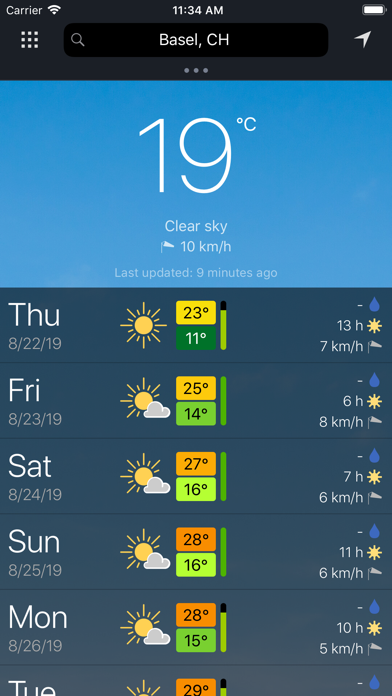A close-up view likely from a tablet screen displays detailed weather information. 

At the top left, the screen shows no cellular bars, indicating the device is connected via Wi-Fi or data. The carrier name is displayed, followed by Wi-Fi signal bars. The time reads 11:34 a.m. On the right, a full battery icon is visible. 

Below, there's a grid of nine dots forming a square, with a search bar featuring the term "Basel, CH." Under this search bar are three dots arranged in a row. The background changes to blue, presenting the weather details in white font: "19 degrees Celsius, clear sky, 10 km/h winds, last updated nine minutes ago."

Transitioning to a dark green-black section, the screen provides extended weather forecasts: 

- On the left, it reads "Thursday 8/22/19: Sunny, high of 23°C, low of 11°C, zero precipitation, 13 hours of sunlight, 7 km/h winds."
- The subsequent line indicates "Friday 8/23/19: High of 25°C, low of 14°C, no rain, 8 hours of sunlight, 6 km/h winds."
- The final entry is for "Saturday 8/24/19: High of 27°C, low of 16°C." 

This detailed weather information helps users plan their days accordingly.